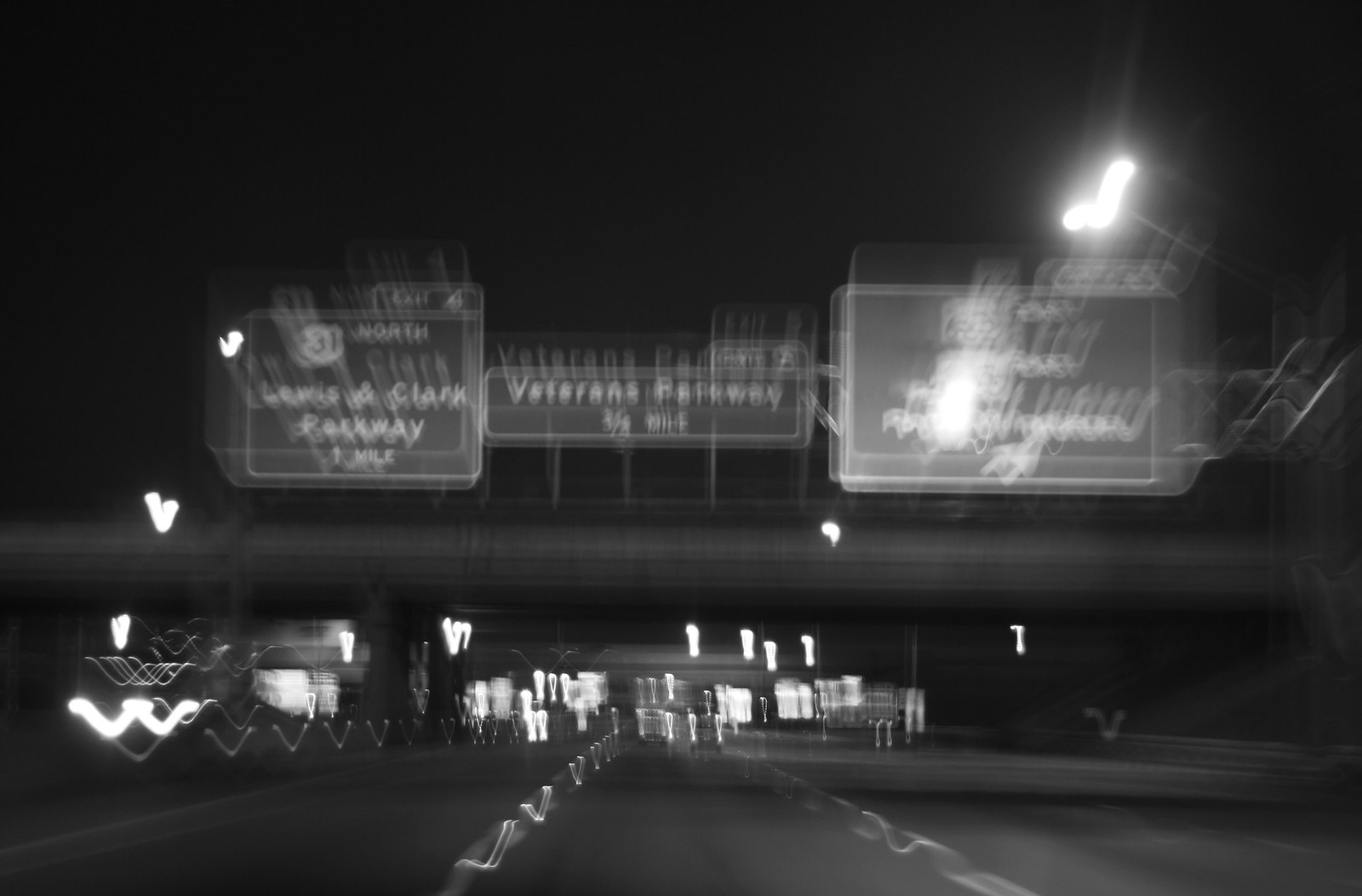This black and white nighttime photograph, taken from the inside of a moving car on the freeway, is notably blurry, suggesting motion and instability. The scene captures a vehicle approaching an underpass, with three large overhead signs marking the structure. The sign on the left reads "31 North Lewis and Clark Parkway, one mile exit forward." The middle sign indicates "Veterans Parkway, three-fourths of a mile" and is smaller in size. The rightmost sign is unreadable due to the brightness of a nearby highway light that washes out the text. The photograph also shows a car driving straight ahead in the distance, and various lights from oncoming traffic creating scattered blurs, contributing to the image's overall sense of movement and lack of clarity.